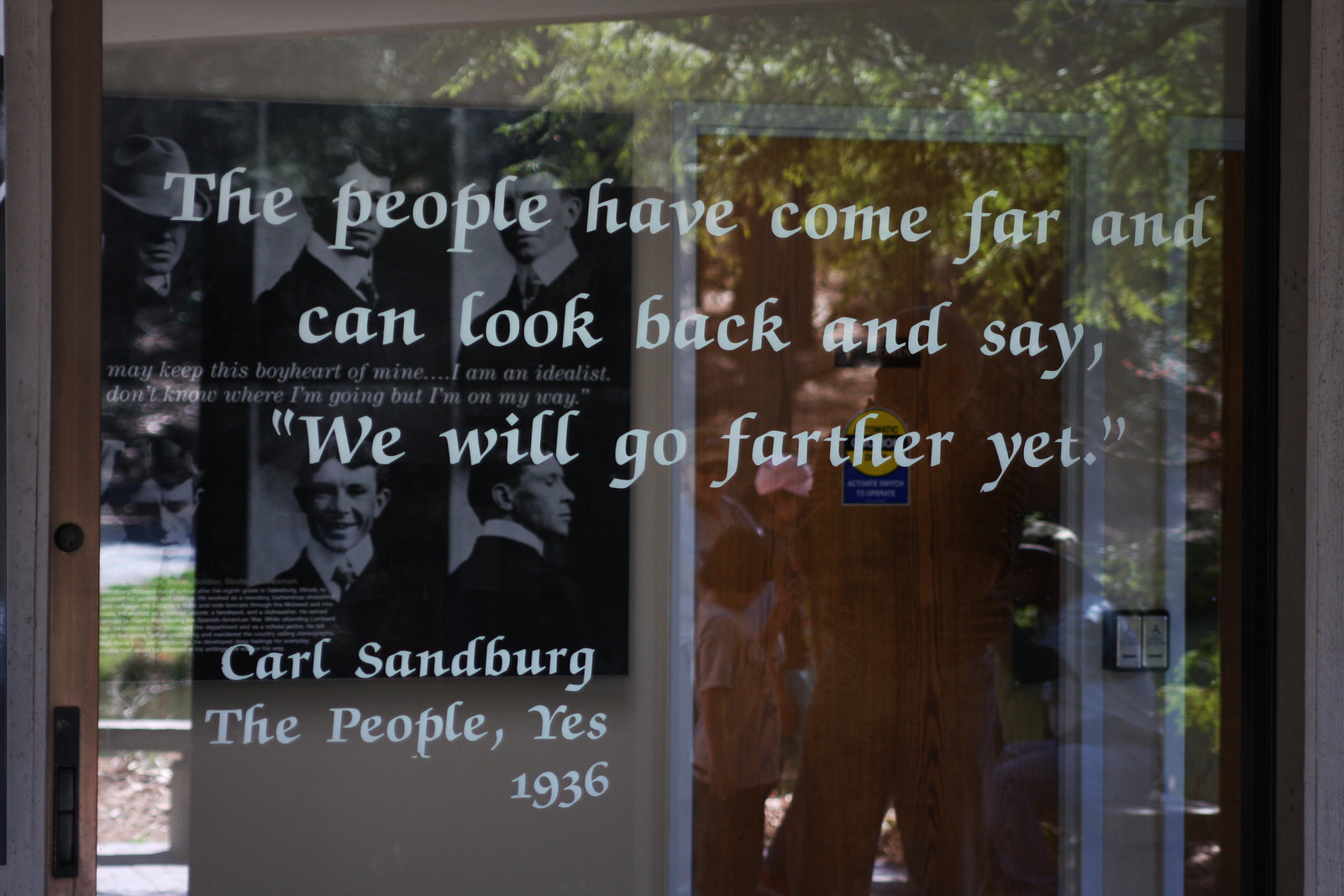This image captures a scene through a glass window adorned with a printed text quote. The quote, in white serif italics, reads: "The people have come far and can look back and say, 'We will go further yet.'" This is attributed to Carl Sandburg, with the citation "The People, Yes, 1936" at the bottom left corner. Through the glass, reflections reveal a park with trees, benches, and several people, possibly including the photographer wearing a beanie. Behind the glass, the interior shows a history exhibit with six black and white profile photos arranged in two rows on the left wall. On the right, there are doors, including a prominent brown door accompanied by a small box near the handle, likely for electronic key access. The window also reflects exterior foliage, adding layers of depth to the image.